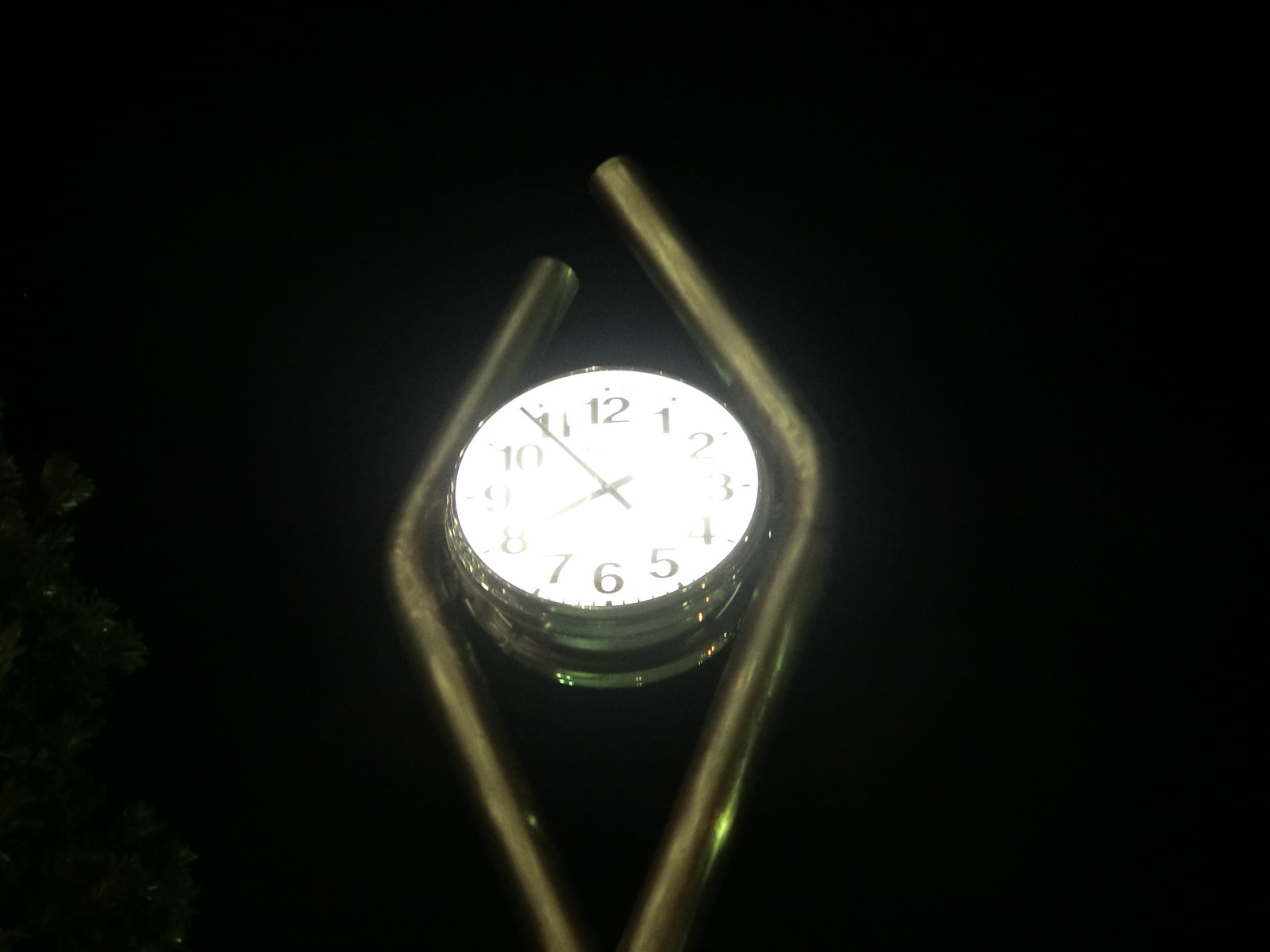This photograph, though slightly blurry, captures a sophisticated timepiece, likely a clock or watch, with a round face adorned with bold Arabic numerals from 1 to 12. The hour and minute hands are clearly visible against the face, providing a classic, functional look. The metal components, predominantly exhibiting a golden, brass-like hue, give the piece a vintage and elegant appearance. The round face is flanked by two diamond-shaped metal arms, extending to the left and right at precise 45-degree angles before converging near the top, though not entirely touching, leaving a small gap. This entire composition is set against a contrasting, pure black background, which further accentuates the intricate details and luxurious color of the metal.